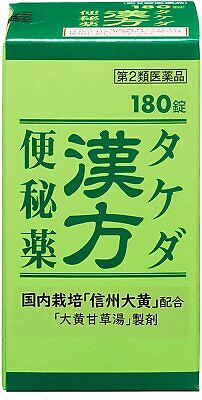The image depicts a green container resembling a juice box, likely made of cardboard, with a mix of two greens: a light green on most of the front and a dark green on the top and edges. The front of the box features predominantly dark green lettering, but some characters are also in black. The writing appears to be in an Asian language, possibly Japanese or Chinese. Notable details include the number "180" on the top right corner and additional, smaller text at the bottom of the label. A white strip, possibly tape, is seen on the top left, suggesting that it might be securing the box. The box is set against a white backdrop.